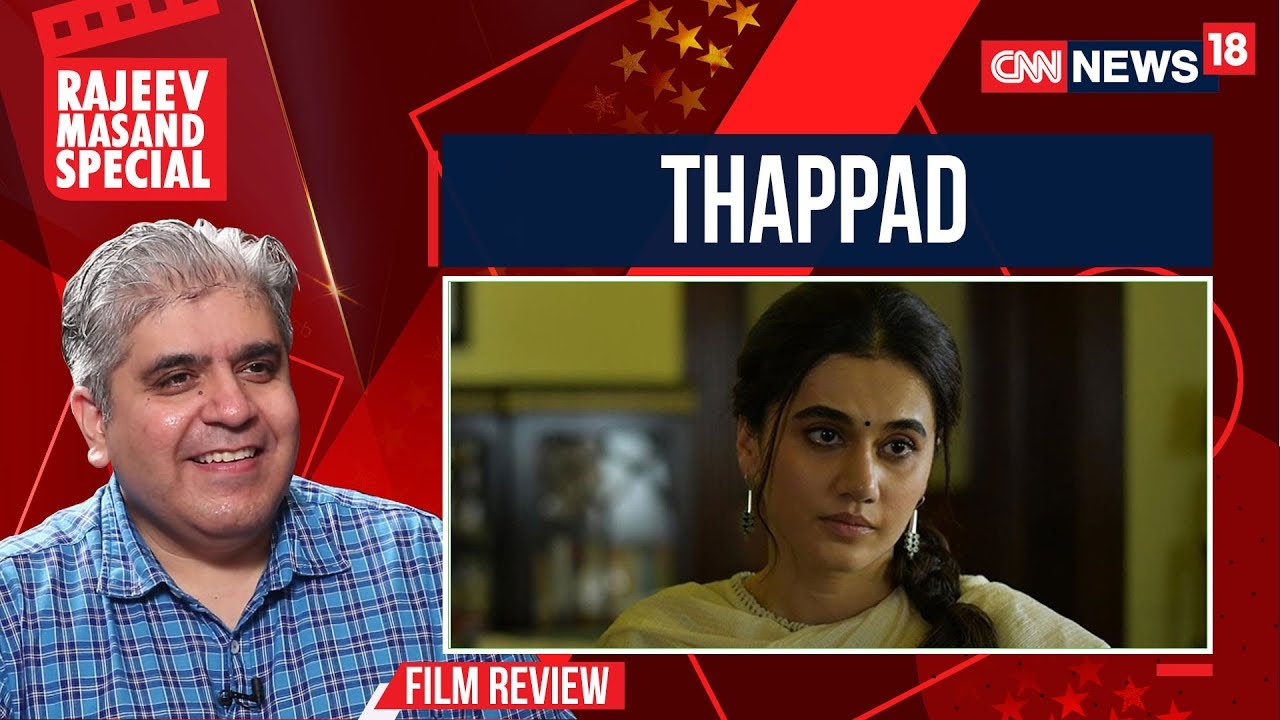The image is a still shot from a CNN News 18 broadcast featuring a film review. On the left side of the screen is Raheem Masand, a film critic, wearing a blue plaid shirt. His name appears in white letters within a red box above his head, labeled as a "Special." The right side of the image shows a woman presented within a white-bordered box; her name, possibly Thapad, is displayed in white letters within a blue box. The background features red tones with gold stars and what seems like a heart. The woman, who appears to be of Hindu ancestry, is wearing a cream swooshy blouse and diamond earrings. Her hair is elegantly tied to the side, and she has a traditional bindi on her forehead. At the bottom of the screen, the label "Film Review" is prominently shown.